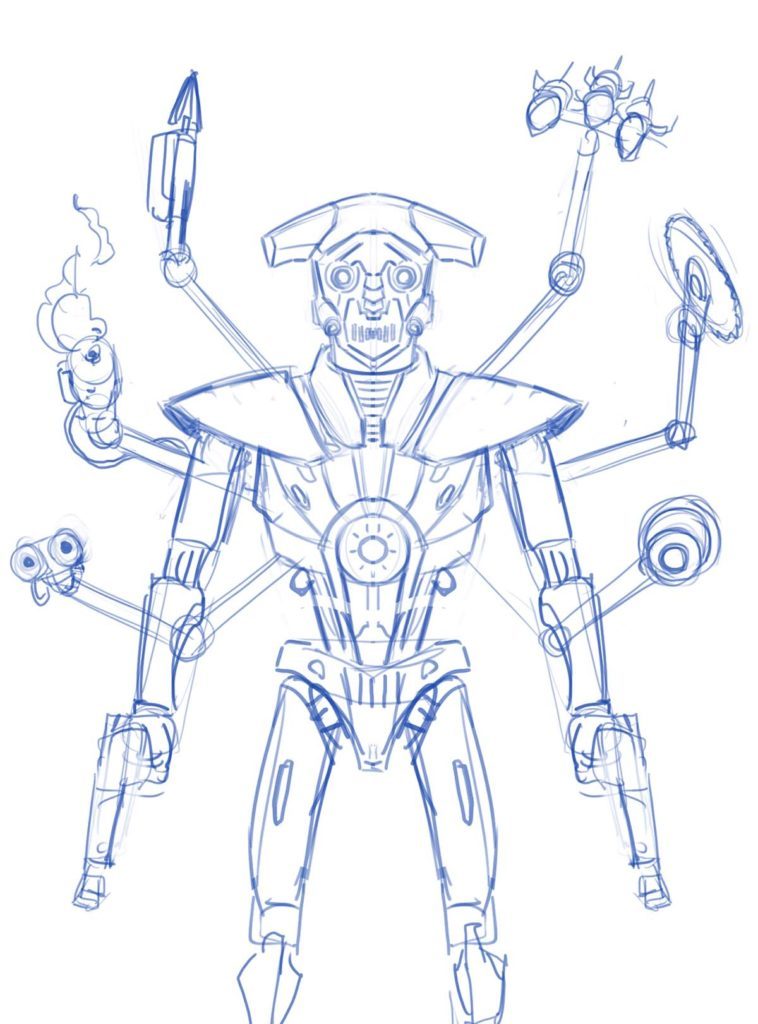This detailed sketch, rendered in blue ink on a solid white background, illustrates a robot-like character with a human-like body and an imposing arsenal of weapons. The robot features a roughly humanoid form with multiple mechanical arms emerging from its back and sides, giving it a total of around eight appendages. Its primary arms each hold a pistol by its sides, while the auxiliary arms brandish an array of weaponry, including a spear or harpoon, a missile launcher, a circular saw, and a hooking shot among other items. The robot's head is adorned with a mask-like visage, circular eyes, and nub-like protrusions akin to sawed-off horns. The torso prominently displays a circular detail reminiscent of Iron Man's arc reactor, emphasizing its mechanical nature. The sketch provides a transparent look at the robot's intricate, uncovered mechanical components, highlighting the detailed design and concept of this formidable character.